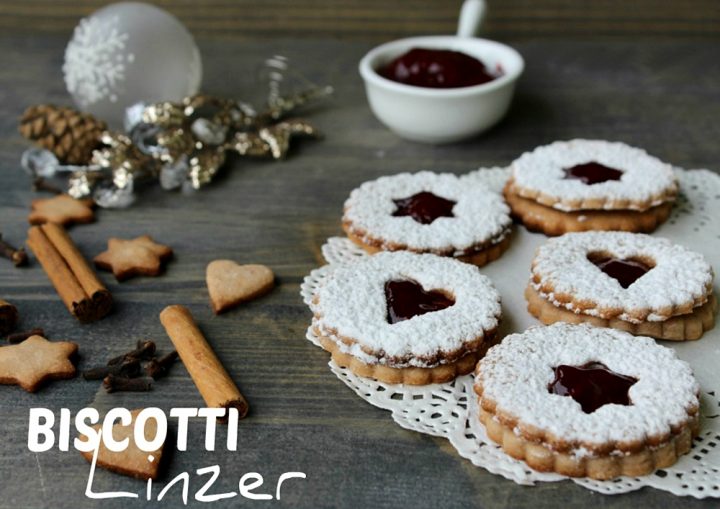The image showcases an assortment of cookies and accompanying decorations artfully arranged on a table. The table features a dark gray surface with light brown or greenish wood grain patterns. In the bottom left corner, white text prominently displays "Biscotti Linzer." A clear, semi-clear plastic bowl filled with red jam and a white spoon is positioned in the top left corner, above a golden decoration with acorns. Below this, there are two cinnamon sticks paired with star-shaped and heart-shaped cookies. The right half of the image is dominated by five sandwich-style Linzer cookies, adorned with white powdered sugar. Each of these cookies features a jam-filled center, with three displaying star shapes and two showcasing heart shapes. They are arranged on a white paper doily. In addition to these, the image includes small pieces of the dough cut out from the cookie centers and miscellaneous decorative elements such as white baubles and nature-inspired adornments in the background. All items are set against a white patterned sheet, completing the festive, rustic presentation.